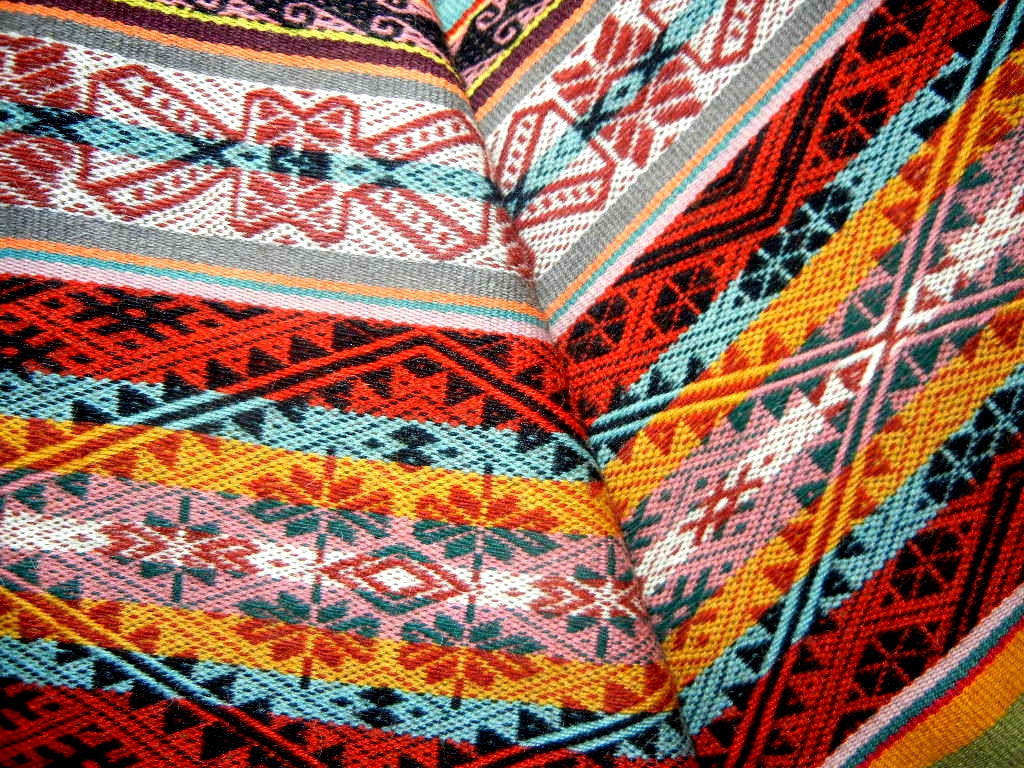This close-up photograph showcases a meticulously hand-woven embroidered piece of cloth, possibly a tapestry or rug, highlighting its intricate design and vivid colors. The cloth is composed of two diagonal pieces stitched together with a seam running from the middle top to the bottom right corner. At the bottom part of the image, a prominent diamond-shaped pattern is featured, surrounded by black or dark blue triangles. Inside the diamond, there are snowflake-shaped chevrons arranged in two rows at the top, three in the middle, and two at the bottom. 

The cloth displays a vibrant spectrum of colors, with stripes of red, light turquoise blue, yellow-orange, pink, and white, repeating in reverse order below. Additionally, in the bottom right corner, a series of green, yellow, red, blue, and white stripes add a burst of color. Above this section, there are alternating stripes in red, green, orange, pink, white, with a unique design comprising thin strips of pink, blue, orange, and gray on a white background with red characters. The top portion of the cloth features a stripe pattern in gray, orange, brown, yellow, and pink.

The design boasts geometric shapes outlined in black, creating a harmonious blend of contrasting colors such as turquoise, blue, orange, yellow, pink, and greens, all finely stitched together. The overall composition is an ordered yet colorful tapestry that reflects both the intricacy of its craftsmanship and the harmony of its vibrant hues.